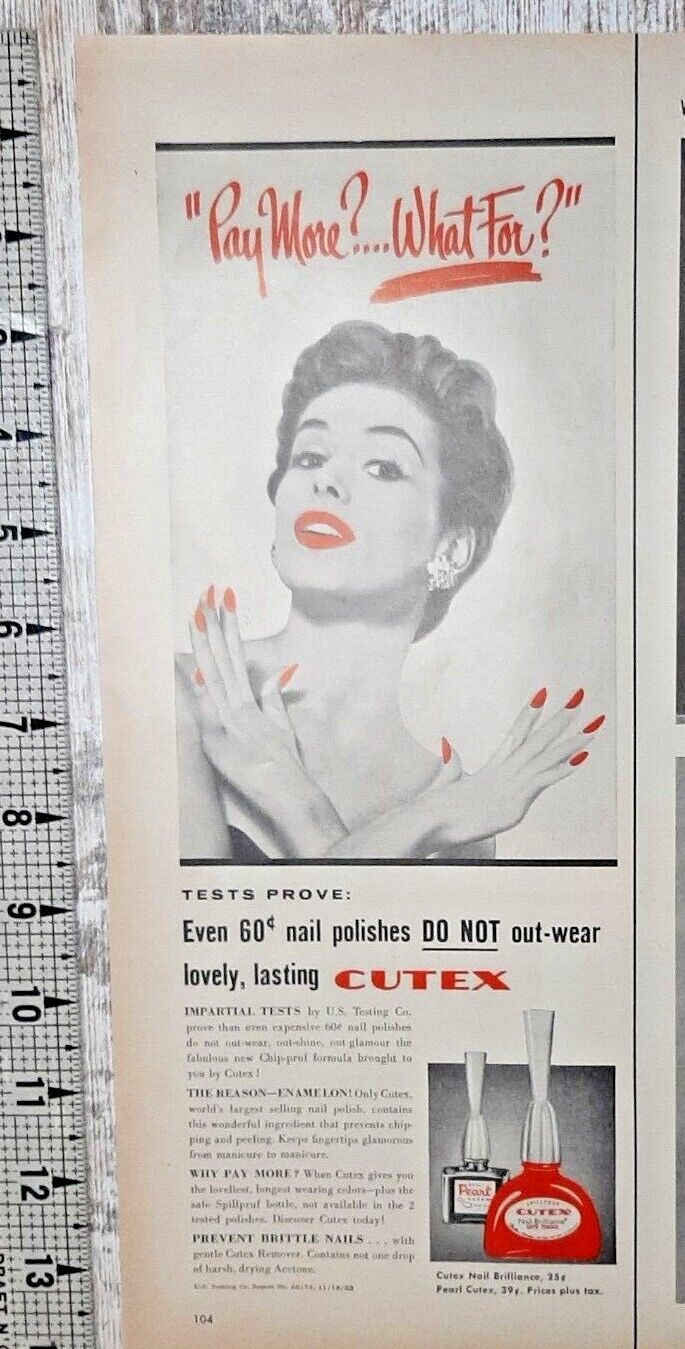This image depicts a vintage advertisement for Cutex nail polish, displayed on a worn white wooden table with a measuring tape along the left-hand side. The advertisement is printed on an aged, slightly orange piece of paper. At the top, bold red cursive text reads, “Pay more... what for?” Underneath, two orange lines emphasize the question. The centerpiece of the ad is a striking black-and-white image of a woman with short, curled hair, adorned with diamond clip-on earrings. Her lips and nails are vividly highlighted in red. She gazes at the viewer, her mouth slightly open, while her arms are crossed at the wrists, showcasing her long, red-painted fingernails. Below her image, black and red text states, "Tests prove even 60 cent nail polishes do not outwear lovely lasting Cutex." Further small, illegible text follows, accompanying an image of a red Cutex nail polish bottle in the foreground, with a likely clear "pearl" polish bottle behind it. This nostalgic clipping evokes the elegance and durability of classic Cutex products.